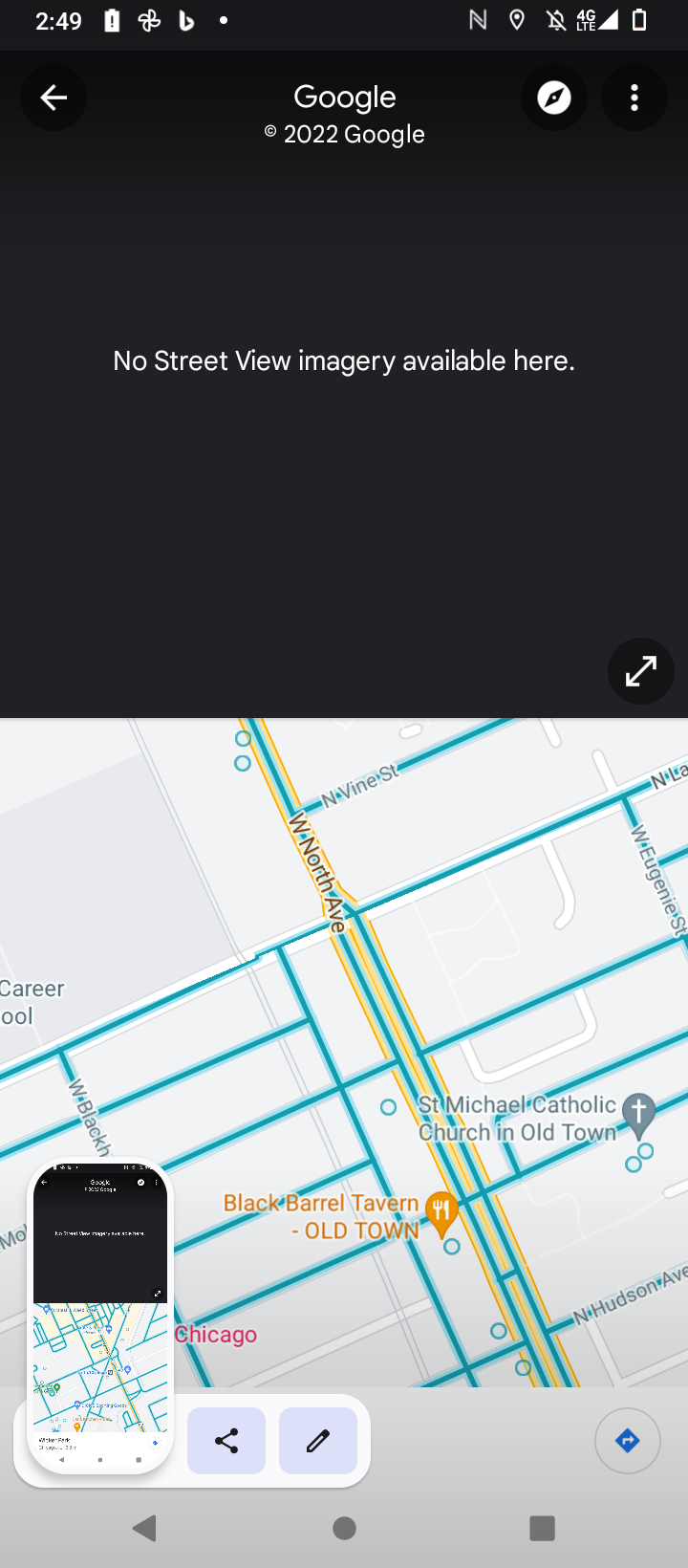The photograph captures the screen of a smartphone, likely cropped for a closer view, depicting a mapping interface. The screen displays a map of Chicago with specific locations such as Black Barrel Tavern, Old Town, and St. Michael Catholic Church in Old Town labeled prominently. The map also highlights streets like North Hudson Avenue, West North Avenue, and North Vine Street, providing a close-up of the city's layout. The upper portion of the screen features a notification with a black background stating, "No street view imagery available here." 

Additional indicators include a timestamp, battery level, and a 4G LTE signal, alongside several buttons and logos, with a "Google 2022" mark, confirming the map's source and date. The lower left corner of the image shows a smaller representation of the smartphone, mimicking the display seen on the main screen, thereby reinforcing that the image pertains to a smartphone.